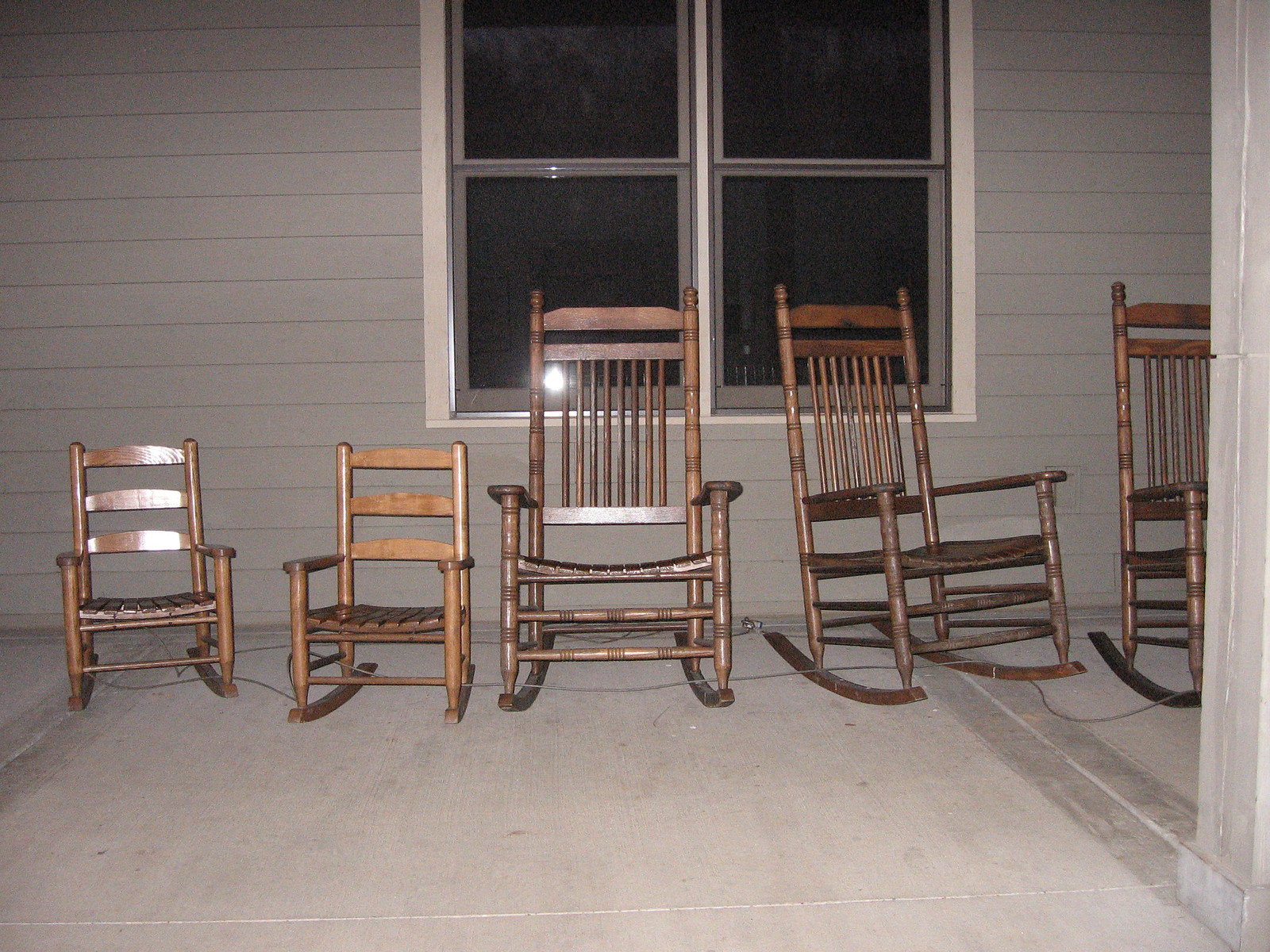This photograph captures a detailed scene of a house's front porch, showcasing a collection of rocking chairs on a gray, shiplap-sided exterior with contrasting white or light tan window trim. The porch itself is concrete, and there are five rocking chairs in total. On the left side, there are two smaller, child-sized rocking chairs, each angled slightly but facing forward. The right side features three larger, adult-sized rocking chairs, with distinct U-shaped bases designed for rocking. One of these larger chairs faces directly forward, while another is angled to the right, and the fifth chair is partially cropped from the image. A concrete pillar stands on the right edge of the photograph, supporting the porch roof. The photograph appears to have been taken with a flash, evident from the reflection in one of the windows, and a security wire is threaded through the chair bases, securing them from theft.